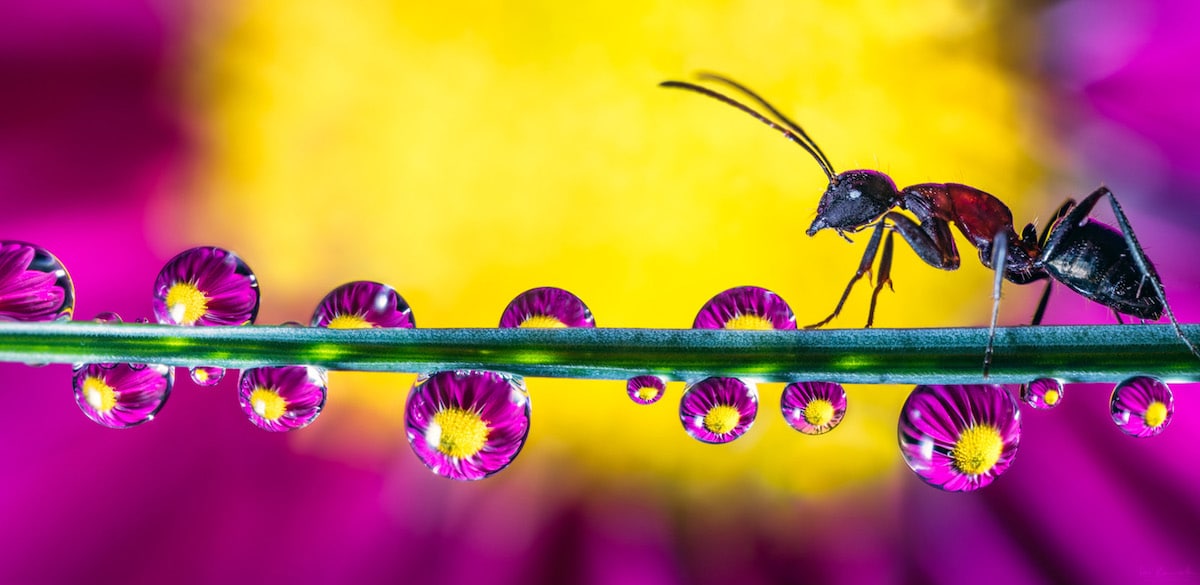In this close-up, highly detailed photograph, an ant with a reddish-brown body and a black abdomen is seen walking along a horizontally laid blade of grass. The ant's long antennae and purplish tint, likely caused by the reflection, add to the image's vivid detail. Surrounding the ant, numerous glistening water droplets—about five on top and ten on the bottom—capture and reflect the background of an out-of-focus flower with striking purple petals and a bright yellow center. Each water droplet presents a slightly different angle of the same flower, creating a mesmerizing array of tiny, refracted images. The blurred backdrop enhances the overall purple glow of the scene, making the pale to green blade of grass on which the ant treks even more striking. The ant is positioned towards the right of the image and is facing left, adding a sense of movement and exploration to this intricate natural tableau.